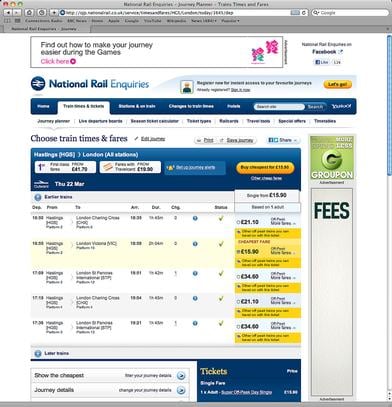The image depicts the National Rail Enquiries interface showing various train times and fares for Thursday, March 22nd. The details are somewhat blurry, making it difficult to read, but some information can be discerned:

1. **Route: London to Vienna**
   - **Departure:** 16:34
   - **Fare:** £18.00
   - **Status:** On time

2. **Route: Hastings to London**
   - **Departure:** Various
   - **Fares:**
     - £21.90
     - £18.51
     - £14.60
     - £21.10
     - £14.40
   - **Status:** All trains are on time
   
Additionally, it mentions that badges are available for purchase from 15.90 pence, which might offer discounted fares for certain routes. The image's poor resolution makes further details hard to decipher.